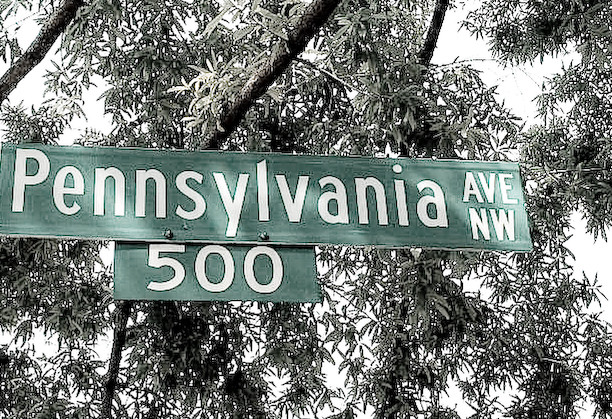In this predominantly black and white photograph, the camera is angled upward, capturing the elements of the scene with dramatic contrast. Central to the image is a street sign, featuring the address "Pennsylvania Avenue, NW" and "500" in a muted white font against a noticeably dull green background. Despite the lack of saturation in the photo, the green hue of the sign remains discernible amidst the grayscale environment. 

The sign comprises two distinct parts: a larger rectangular top piece displaying "Pennsylvania Avenue, NW" and a smaller rectangular piece below it showing "500". The background is filled with the stark silhouette of tree branches and leaves, which are rendered in shades of black and white. These branches and leaves spread across the scene, with pockets of white sky peeking through, adding depth and texture to the otherwise monochromatic backdrop. The leaves are variously described as broad and thin-edged, resembling those of an oak tree. Three structures, possibly trunks or ropes, descend diagonally across the photograph, contributing to the dynamic composition of the image, while the background of the sky seems overcast, appearing gray and somewhat cloudy.

This deliberate interplay of shades and the eerily preserved color of the street sign create a hauntingly captivating scene that draws the viewer's gaze directly to the iconic address.